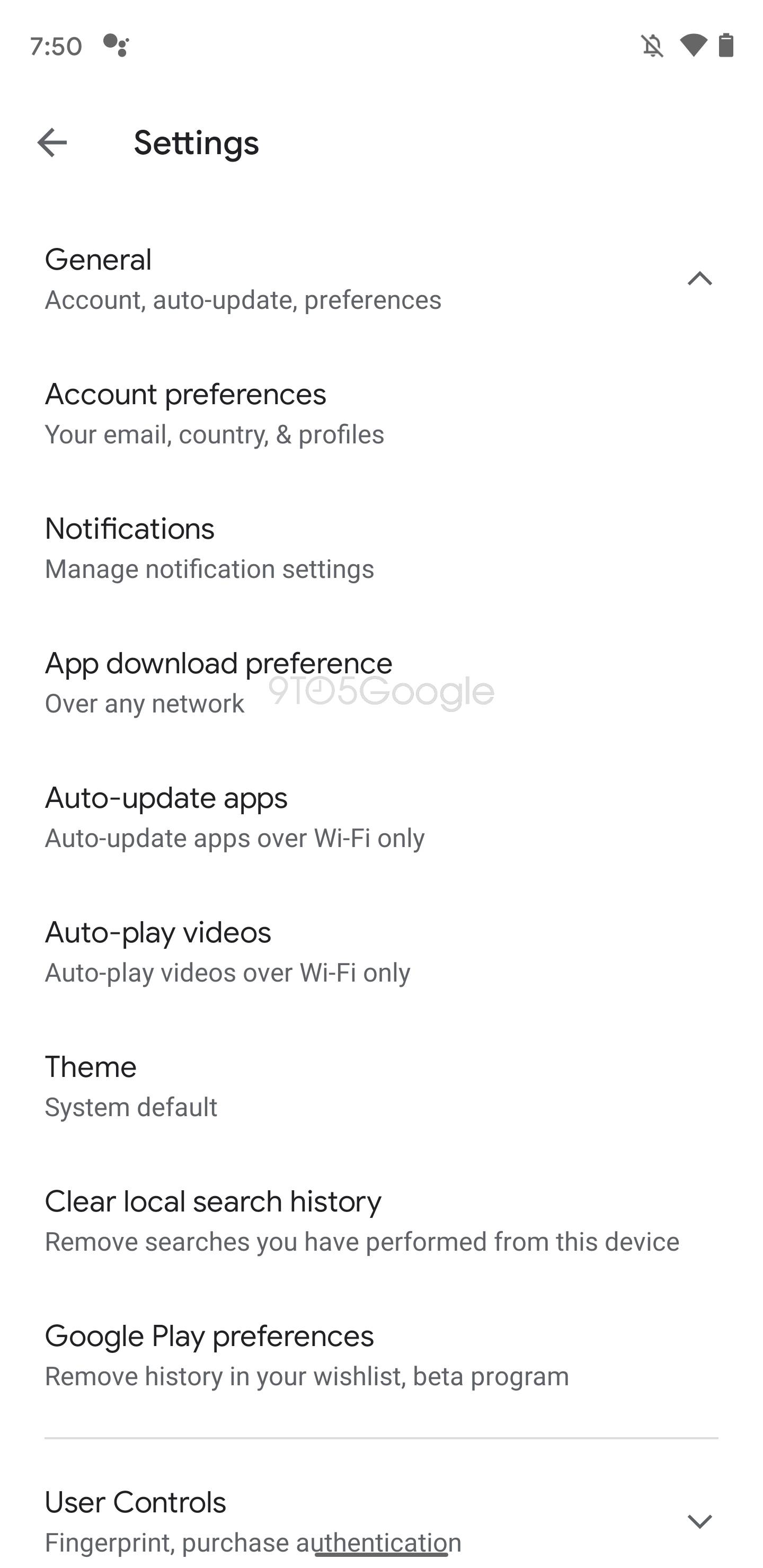In this image, there is a screenshot of a mobile device displaying a settings menu. 

**Top of the Screen:**
- **Left Corner:** The time is displayed as 7:50.
- **Right Corner:** Icons for notifications, Wi-Fi connectivity, and battery level are visible.

**Menu Layout:**

1. **General Section:**
   - **Accounts**
   - **Auto-Updates**
   - **Preferences**

2. **Account Preferences:**
   - **Your Email**
   - **Country**
   - **Profiles**

3. **Notifications:**
   - **Manage Notification Settings**

4. **App Download Preference:**
   - **Over Any Network**

5. **Auto-Update Apps:**
   - **Auto-Update Apps Over Wi-Fi Only**

6. **Auto-Play Videos:**
   - **Auto-Play Videos Over Wi-Fi Only**

7. **Theme:**
   - **System Default**

8. **Clear Local Search History:**
   - **Removes Searches You Have Performed From This Device**

9. **Google Play Preferences:**
   - **Remove History From Your Wish List**

10. **Beta Program**

11. **User Controls:**
    - **Fingerprints**
    - **Purchase Authentication (Repeated multiple times)**